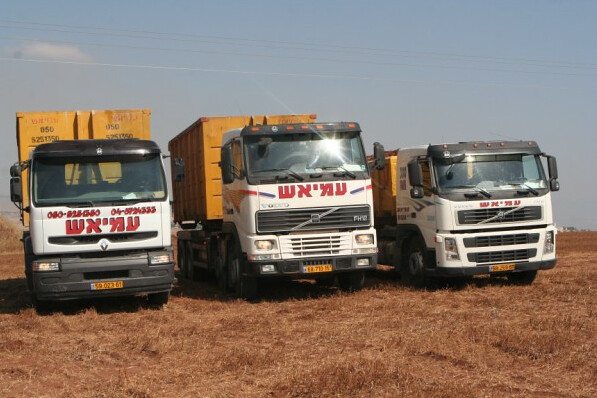In the image, three white trucks of varying sizes are parked on a patch of brownish, straw-like grass. The trucks, belonging to the same company, each have red lettering on the front; the truck on the far left also displays a phone number above the red lettering. The trucks, aligned side by side, carry orange cargo containers on their backs. The smallest truck is on the right, with cargo that doesn't rise above its lower cab, while the largest truck is in the middle, bearing cargo that extends above its taller cab. The third truck, the one on the left, has cargo that appears even taller than the middle truck’s. Power lines hang overhead, and a clear blue sky features a single white cloud in the upper left corner. Distant structures hint at civilization beyond the field. The sun shines brightly, casting a well-lit scene despite one person perceiving a slightly gray sky.